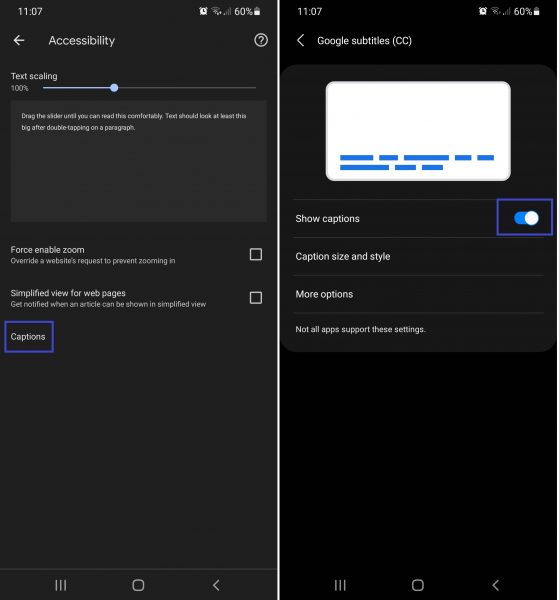Here are two detailed captions for the given images:

**Left Image Caption:**

The left image shows a cell phone or tablet screen at 11:07 AM, as indicated by the time display at the top of the screen alongside an alarm clock icon, a 60% battery indicator, and Wi-Fi symbols. Below the status indicators, there is a row of icons and text on a black background featuring a left arrow, an accessibility icon, and a question mark enclosed in a circle on the far right. Below that, text reads "Scaling 100%" accompanied by a sliding bar positioned about one-third of the way to the right. The instruction, “Drag the slider until you can read this comfortably. Text should look at least this big after double tapping on a paragraph,” follows. Further down, there are two settings options: “Force enable zoom, overtake a website's request to prevent zooming in,” and “Simplified view for webpages, get notified when an article can be shown in a simplified view,” both with unchecked checkboxes next to them. The word "Captions" is highlighted inside a blue box. At the bottom of the image, the navigation icons include three vertical lines, a square, and an arrow pointing to the left.

**Right Image Caption:**

The right image, also with a black background, displays the same status indicators at the top: the time 11:07 AM, an alarm clock icon, a Wi-Fi signal, and a 60% battery indicator with its icon. Below that, a left-pointing arrow is labeled "Google subtitles (CC)." A white box contains two rows of blue horizontal lines of varying lengths at the bottom of the box. Below this, a row labeled “Show captions” displays a blue toggle switch flipped to the right, indicating that captions are turned on. The next row labeled “Caption size and style” suggests there are further customization options available, though not all apps support these settings. Similar to the left image, the bottom of the screen features three vertical lines, a square, and an arrow pointing to the left, representing the navigation icons.